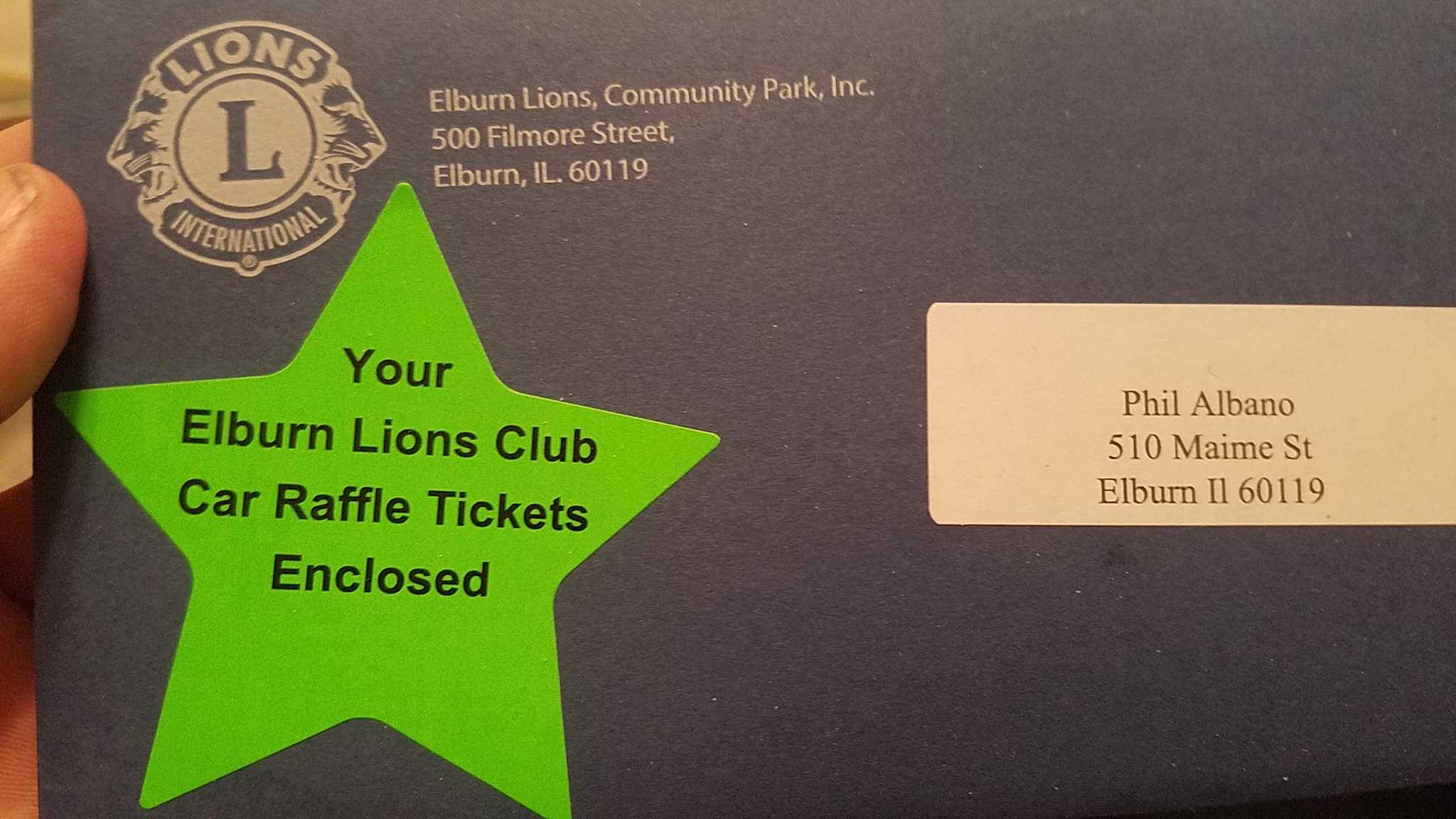The image showcases a dark gray envelope from the Elburn Lions Community Park, Inc., located at 51500 Fillmore Street, Elburn, Illinois, 60119. In the upper left corner, there's an emblem of Lions International, featuring a central "L" flanked by lion heads on either side of the crest. To the right of the emblem, the return address is written in yellowish print. The envelope is addressed to Phil Albano at 510 Main Street, Elburn, Illinois, 60119. On the left bottom side, a prominent green star with black text announces, "Your Elburn Lions Club Car Raffle Tickets Enclosed." On the right side of the envelope is a tan-colored rectangle with the recipient's address. Additionally, you can see a person's thumb peeking from the left edge of the image, holding the envelope.